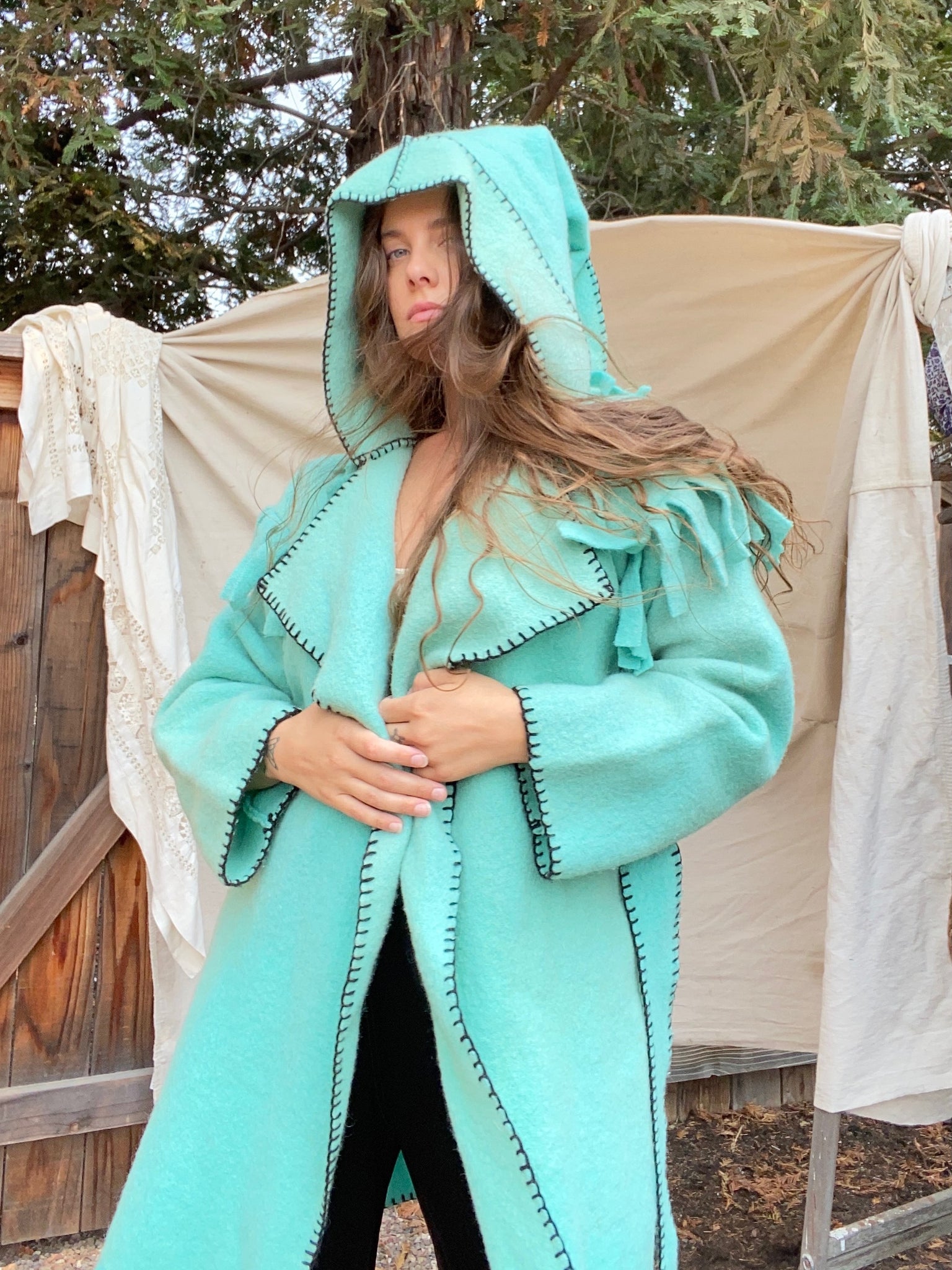In this color photograph, a young woman in her mid-twenties stands outdoors, framed by a backdrop of nature and rustic elements. She is positioned in front of what appears to be a wooden gate, draped with a canvas-like cloth that features delicate lace detailing. A large green tree can be seen in the background, although it is mostly obscured by the sheet.

The woman has long, light brown hair that reaches nearly to her elbows and is caught slightly by the wind, adding motion to the scene. She gazes directly at the camera with a serious, almost defiant expression in her striking bluish-gray eyes. She is dressed in a mint green, felt-like hooded coat that has distinct black whipstitching around the seams and edges. The coat has wide lapels and a subtle fringe around the collar and shoulders, lending it an unusual texture. It appears she is either holding the coat closed across her midsection or is in the act of opening it, revealing a glimpse of black pants beneath.

The rich details of her attire and the setting—a clash of the natural and the crafted—create a vivid, contemplative image.